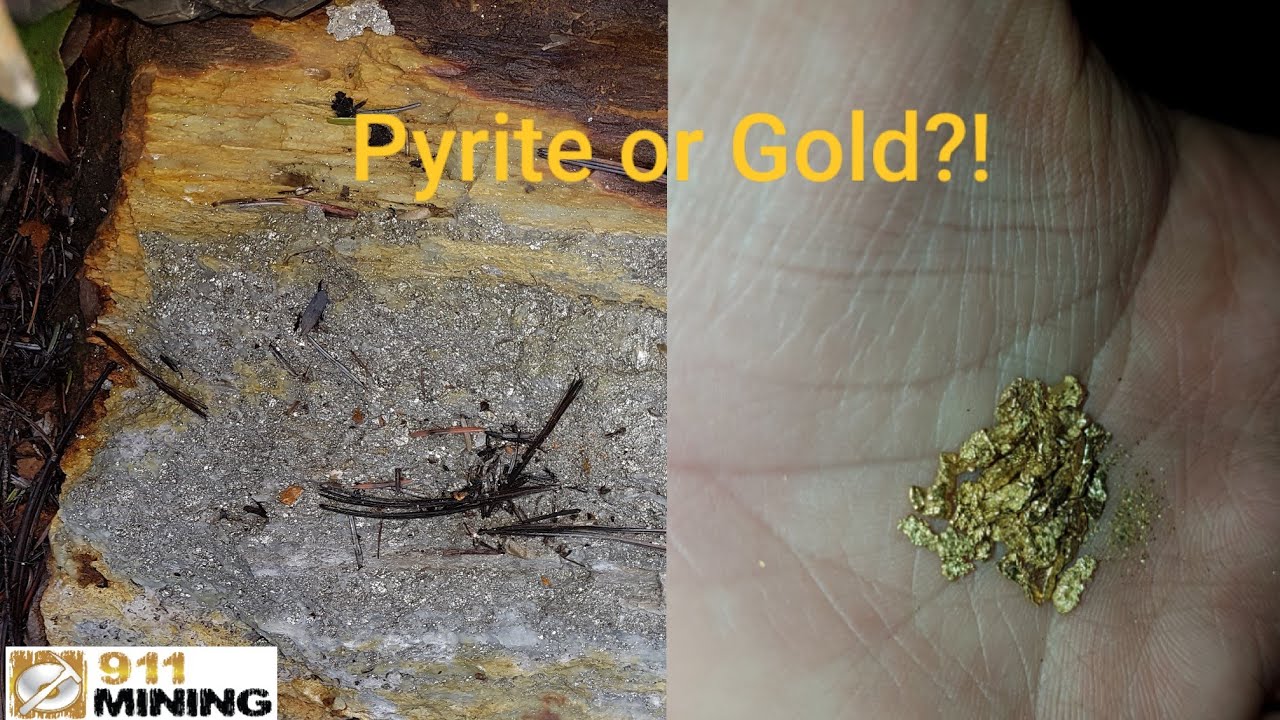A detailed caption for the image could be:

"The rectangular image is composed of two separate color photographs displayed side-by-side, each occupying 50% of the overall space. Across the top center, bold gold lettering reads 'Pyrite or Gold!?' Intricately designed, the photograph on the left showcases a fragment of gold-colored rock adorned with silver-like material, described by some as a mixture of beige dust with embedded twigs, resembling tiny rocks glued together with a wooden border. In juxtaposition, the right photograph visually captures the upturned palm of a hand, meticulously displaying a small pile of gold flecks nestled within its lines. Enhancing the theme with a touch of realism meets graphic design, the bottom left corner features a white horizontal rectangle showcasing a gold square logo illustrated with a silver bowl and hammer. Adjacent to this logo, gold and black text reads '9-1-1 Mining.'"